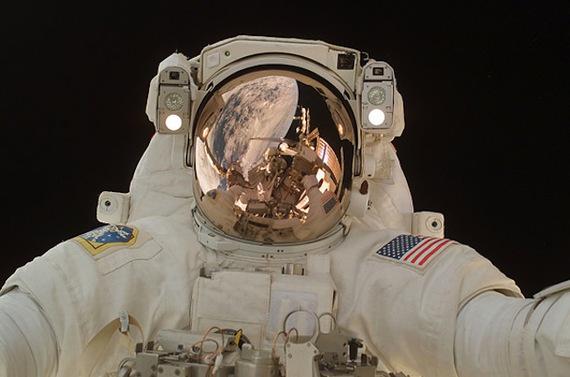The photograph captures a lone astronaut in outer space, clad in a heavy, white spacesuit adorned with an American flag patch on one arm. The astronaut, holding out both hands, appears to be taking a selfie with a large, bulky camera. Mounted on each side of the helmet are illuminated lights and cameras. The reflective visor, displaying a mirror-like and slightly sepia-tinted surface, reveals distorted images of Earth, some nearby equipment or spacecraft, and the vastness of space behind the astronaut. The background is a deep black, punctuated by faint, distant stars. The astronaut is tethered to what seems to be a space station or satellite, emphasizing the isolation and grandeur of the scene.